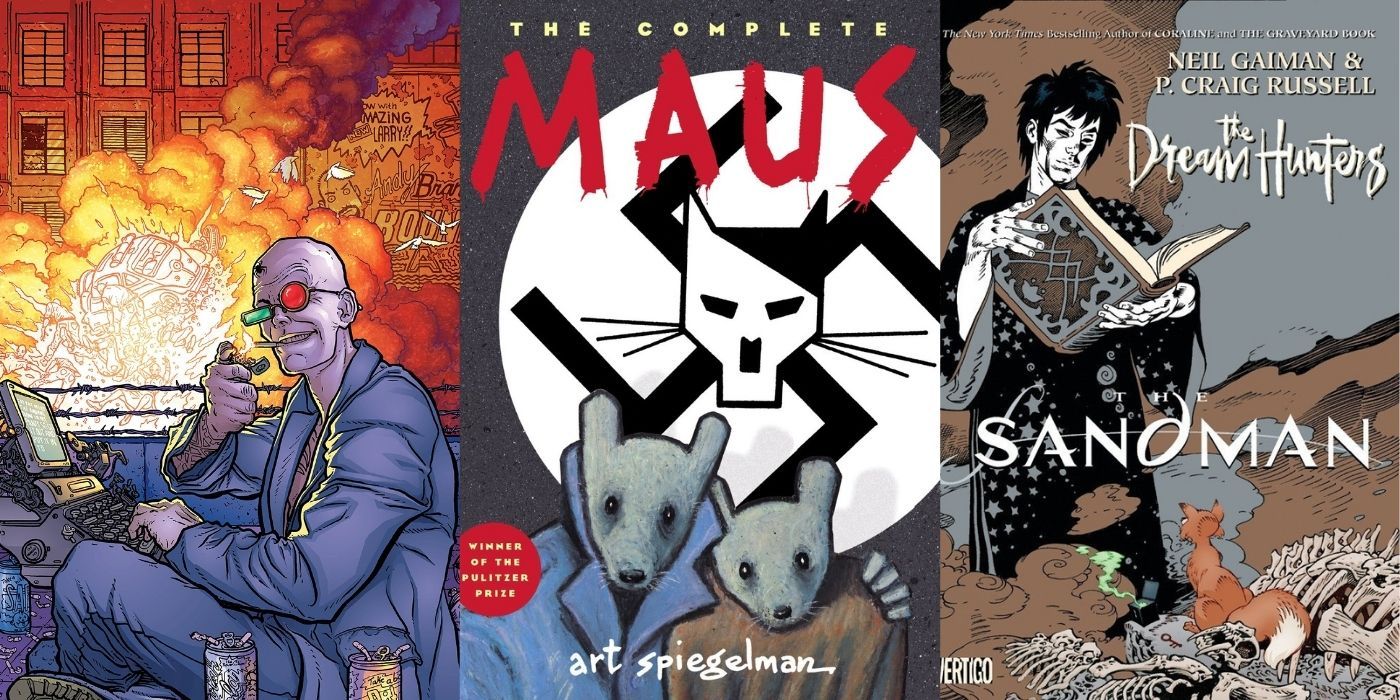Displayed in the image are the covers of three graphic novels arranged in a row. The first cover, from an unidentified graphic novel, features a character with purple skin sitting at a typewriter. He is lighting a cigarette dangling from his mouth in the midst of a dystopian scene, complete with an explosion in the background. The second cover is from the renowned graphic novel "Maus." Prominently displayed is a Nazi swastika, featuring an evil, Hitler-inspired cat at its center, with two mice positioned below. The final cover is from "The Sandman: The Dream Hunters." It depicts a man draped in a long black robe, engrossed in reading a book while surrounded by scattered bones.